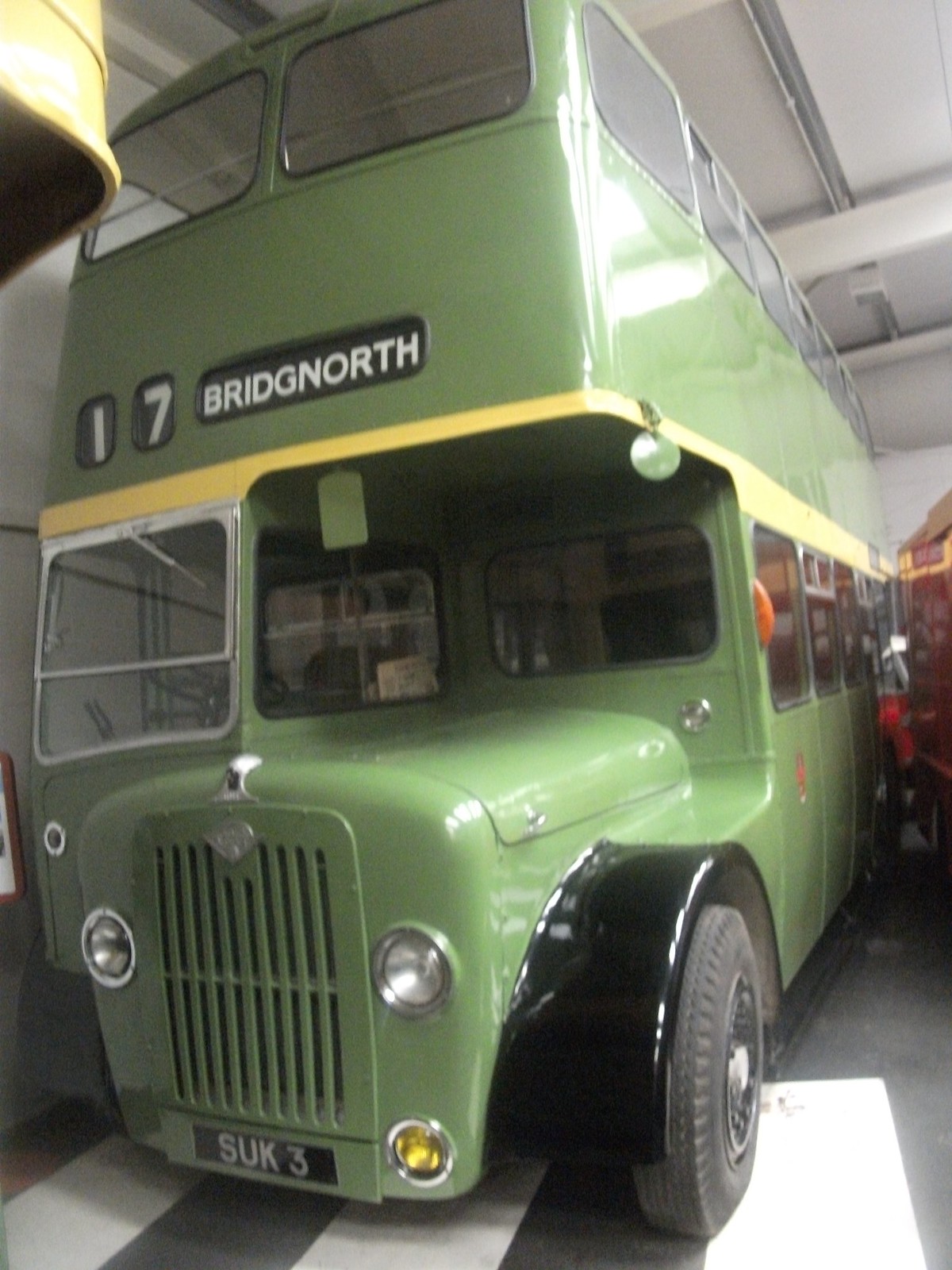The image captures a pristinely restored classic double-decker bus, likely a museum piece, situated seemingly inside a garage or warehouse. The bus, reminiscent of iconic English tourist buses, is adorned in a pastel or olive green color with a distinctive yellow stripe separating its upper and lower decks. It bears a black license plate reading "SUK 3" and features yellow fog lights flanking the plate. The driver's cockpit prominently extends along the side of the engine bay, and above the windshield, the signage displays the number "17" with the destination "Bridge North." The bus rests on black wheel covers, and a crosswalk paint adorns the floor beneath it. To the right, the corner of a red vehicle is visible but not fully in frame, while an additional yellow vehicle is partially visible in the background, further hinting at the confined storage space.